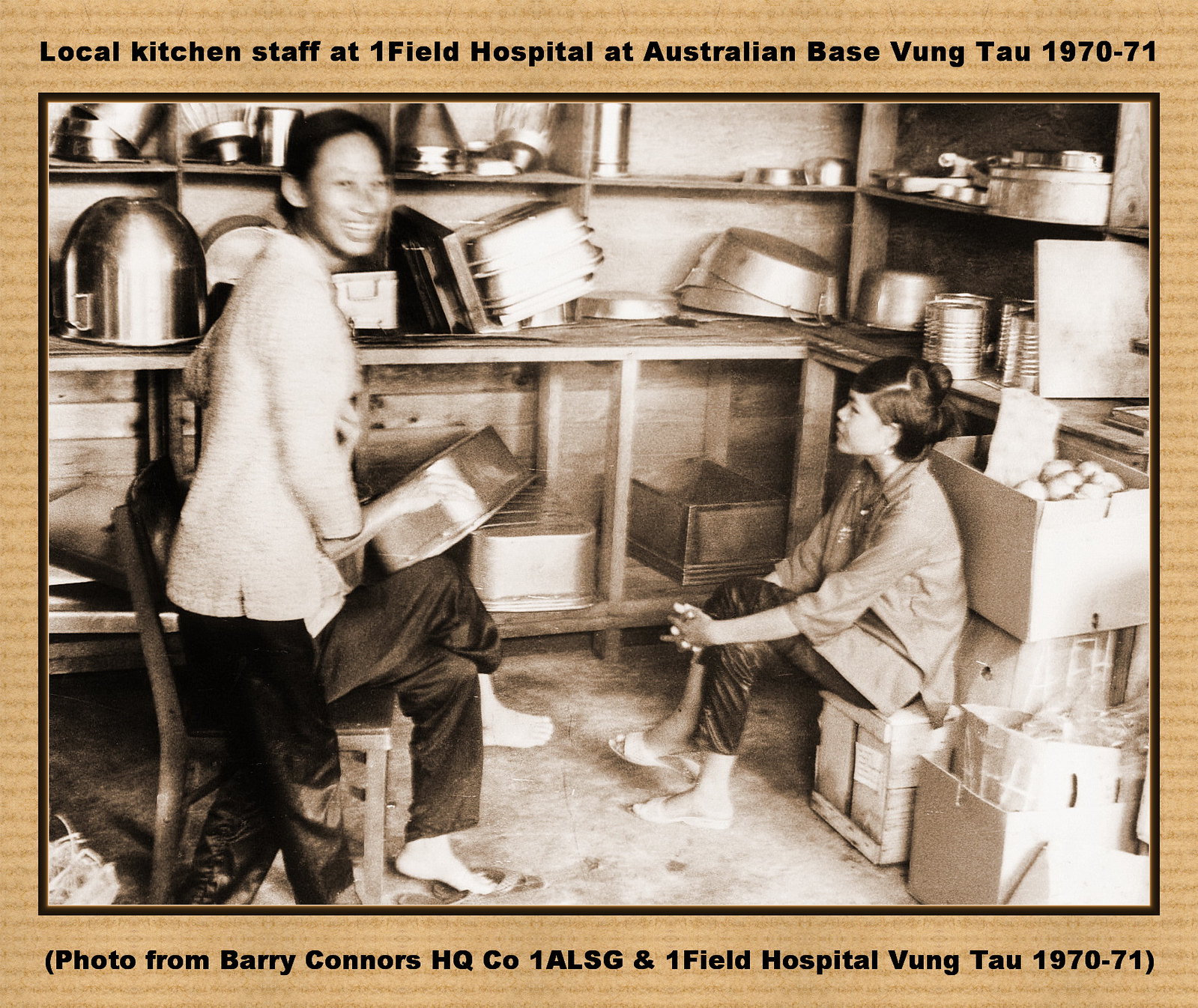This sepia-toned photograph captures an indoor kitchen setting, bordered by a beige frame. The top of the photograph bears the text, "Local Kitchen Staff at Onefield Hospital at Australian Base, Vung Tau 1970-71," while the bottom reads, "Photo from Barry Connors HQCO 1ALSG and Onefield Hospital, Vung Tau 1970-71." The image showcases kitchen staff at the Onefield Hospital in Vung Tau, Vietnam, during the early 1970s. On the left, a woman stands smiling, holding a pan. To her right, a young girl with short hair sits on a box, wearing flip-flops. Behind them are shelves lined with numerous stainless steel cooking pans, underscoring the kitchen environment. The photograph exudes a sense of camaraderie and historical ambiance, capturing a moment in time from the Australian base's everyday life.